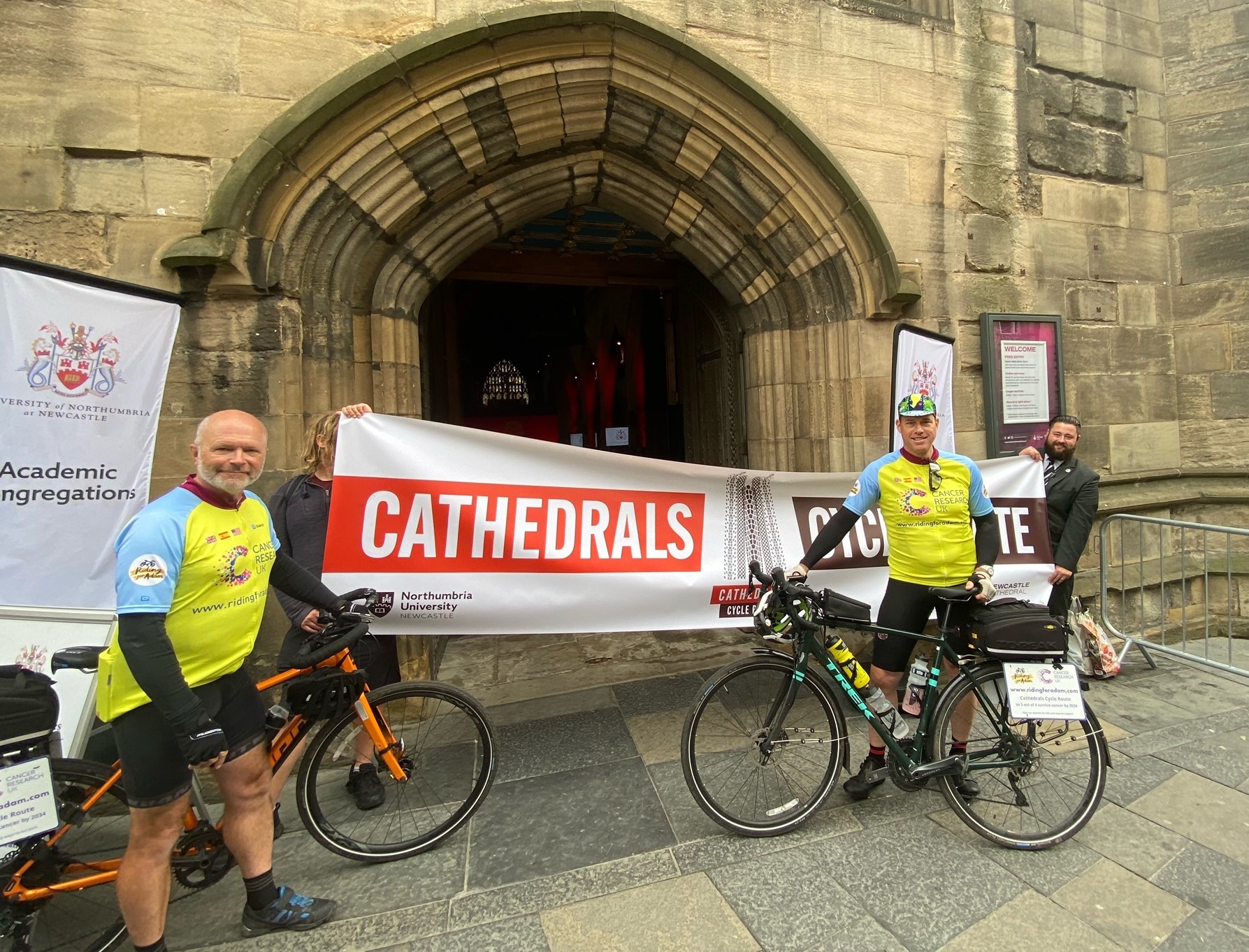In the color photograph, two white male cyclists pose with their bicycles in front of a pebble-stone building featuring a large archway and tiled flooring, likely the entrance to a cathedral. The cyclists, both wearing neon yellow shirts with blue sleeves, black long undershirts, black cycling shorts, and bike shoes, stand with their bikes—one orange and one black. The man with the orange bike is bald with a white beard, while the man with the black bike smiles beneath his helmet. A white banner, held by two additional individuals—a man in a suit with black hair and beard on the left and a partially visible woman on the right—stretches across the archway. The red box on the banner prominently displays the word "Cathedrals" in white letters. The scene suggests the completion of a cycling event or race, possibly in a European location noted for its architectural history.